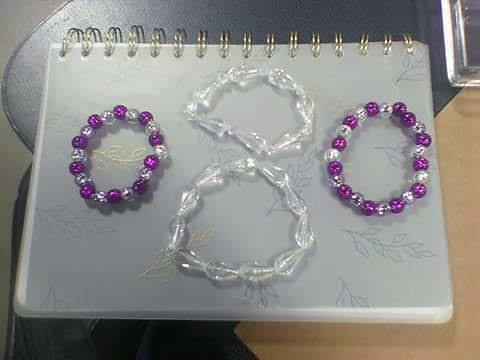The image is a color photograph taken in landscape orientation, capturing a gray spiral-bound notebook, positioned with its spiral along the top edge. The notebook's translucent gray cover features a floral design with thin stalks and leaves drawn in gray pencil, some with reflective gold accents, particularly over the left bracelet. On top of the notebook, which serves as the backdrop, are four beaded bracelets. The two outer bracelets, placed on the left and right, are identical, composed of alternating round white pearlescent and lilac beads. Centrally placed and forming a figure-eight shape, are two wider bracelets with clear, pear drop-shaped crystals. The photograph, slightly low in quality and slightly blurred, also hints at the setting, with a blue chair visible in the left corner and possibly a beige table in the background, along with what appears to be a faint outline of a crystal-clear handle.